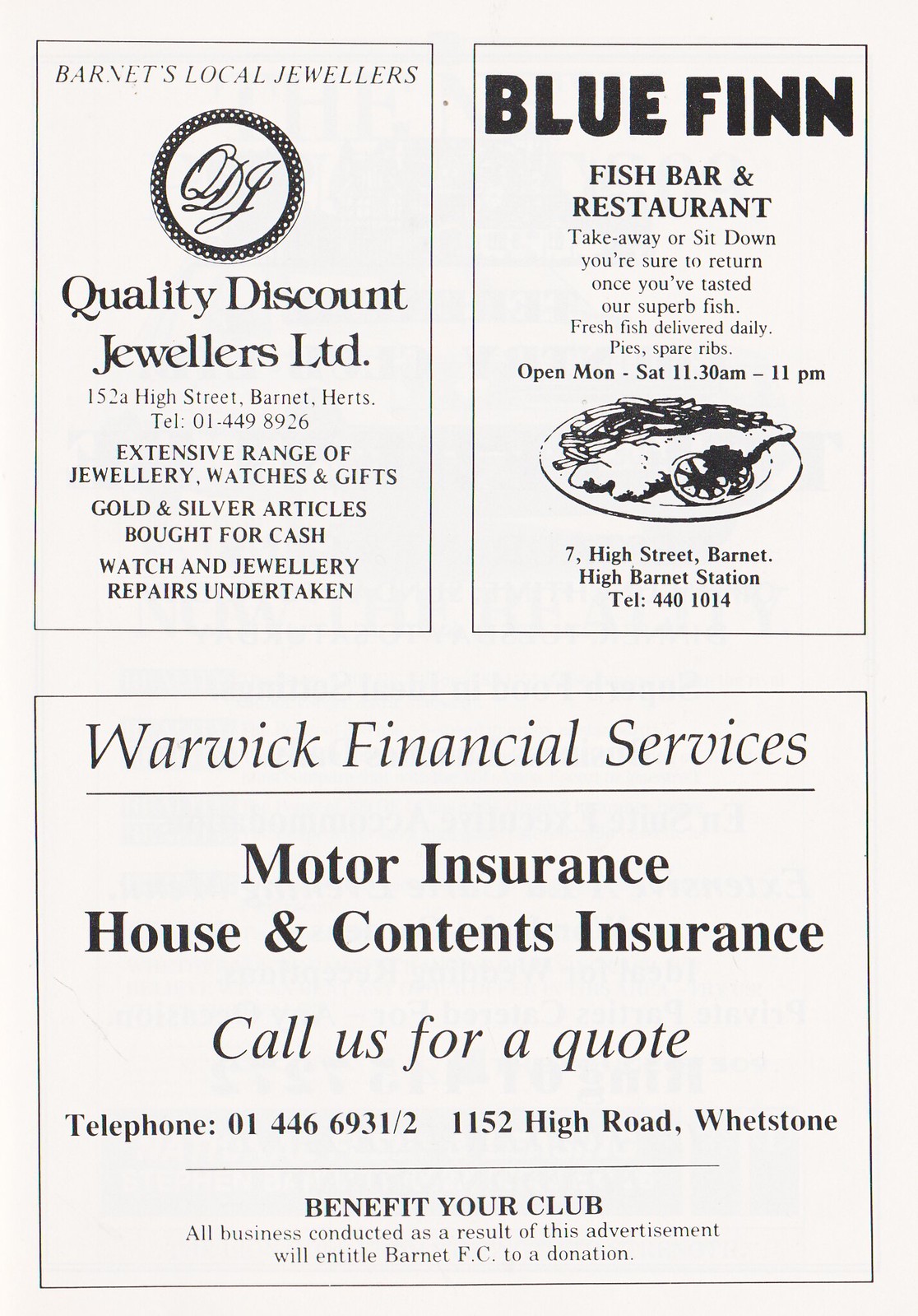The image is a vintage-style black and white advertisement page, divided into three distinct sections, each promoting a different business. 

In the upper left quadrant, it features an ad for Quality Discount Jewelers Limited with their logo—a circle with a frill design enclosing the initials QDJ in cursive. The address, 152A High Street, Barnett Hertz, and contact number, 01-449-8926, are prominently displayed. The jeweler's ad boasts an extensive range of jewelry, watches, and gifts, alongside services such as buying gold and silver articles for cash and undertaking watch and jewelry repairs.

The upper right section advertises the Blue Fin Fish Bar and Restaurant in bold black letters. Below, it highlights the amenities offered: eat-in or takeaway options, with promises of superb fish and fresh daily deliveries. The restaurant, located at 7 High Street, Barnett, near High Barnett Station, operates from Monday to Saturday, 11:30 a.m. to 11:00 p.m. A drawing of a plated fish dish complements the text. The contact number is 440-1014.

The lower half of the page is dedicated to Warwick Financial Services, emphasizing motor insurance, house and contents insurance, and providing quotes. The advertisement includes their contact information, Telephone 01-446-6931/2, and their address, 1152 High Road, Whetstone. At the bottom, it mentions that any business resulting from this advertisement will benefit Barnett FC with a donation.